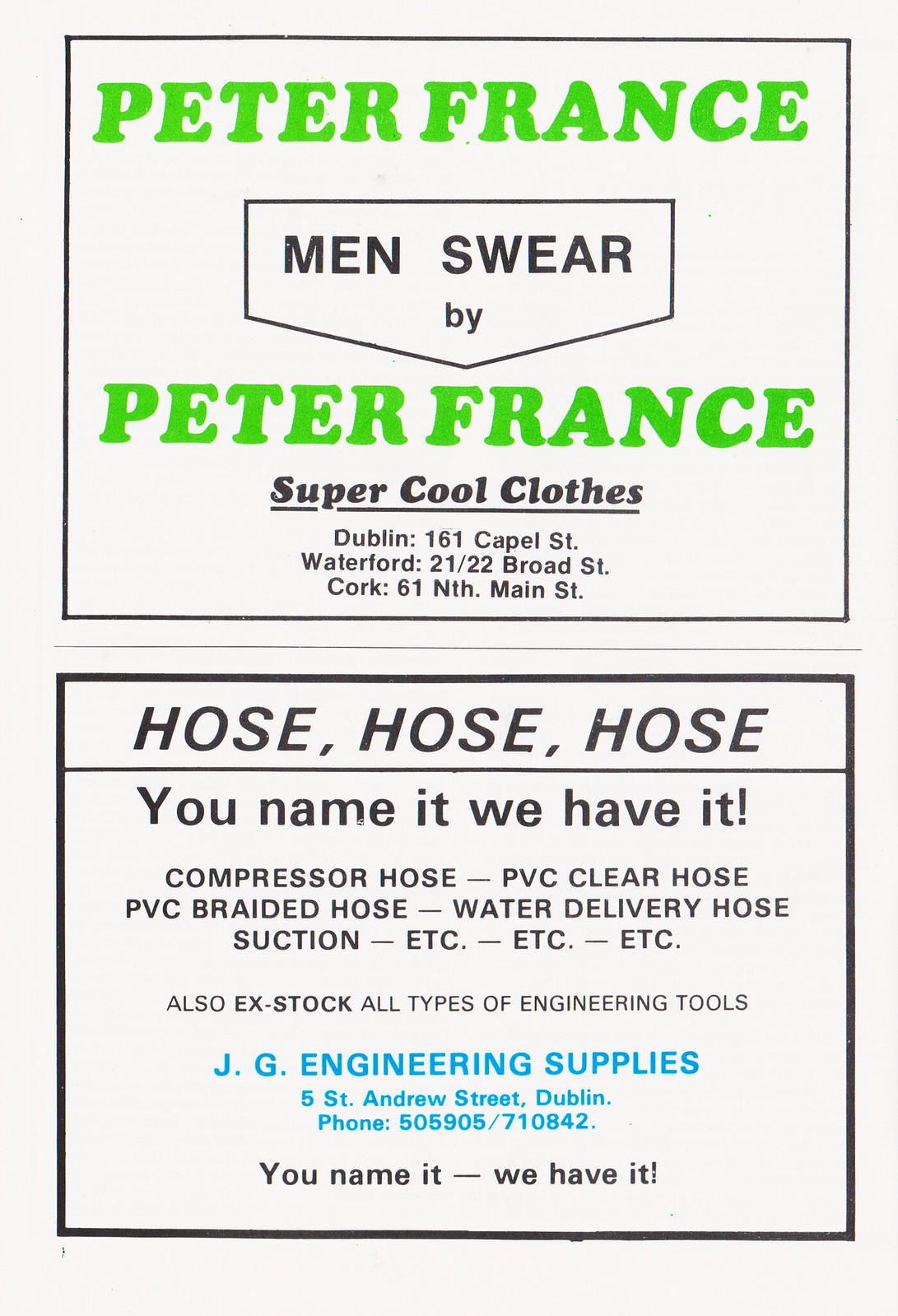This image displays two distinct advertisements on a white background. The first ad, framed within a black-outlined, home-plate-shaped box, features the name "Peter France" in prominent green and black lettering. This section promotes men's fashion, specifying "Men Swear By Peter France – Super Cool Clothes" and lists store locations in Dublin (161 Chapel Street), Waterford (21-22 Broad Street), and Cork (61 North Main Street).

Below the Peter France ad, the second advertisement also has a white background with a black border. It begins with the phrase "Hose, Hose, Hose" and the tagline "You name it, we have it." This section highlights various types of hoses including compressor hose, PVC clear hose, PVC braided hose, water delivery hose, and suction hose, followed by the phrase "etc, etc, etc". Additional offerings include "X-stock – all types of engineering tools." The ad concludes with the business name "J.G. Engineering Supplies," given in blue lettering along with the address "5 St. Andrew Street, Dublin" and the phone number "505-905-710842." The repeated slogan "You name it, we have it" underscores their comprehensive inventory.